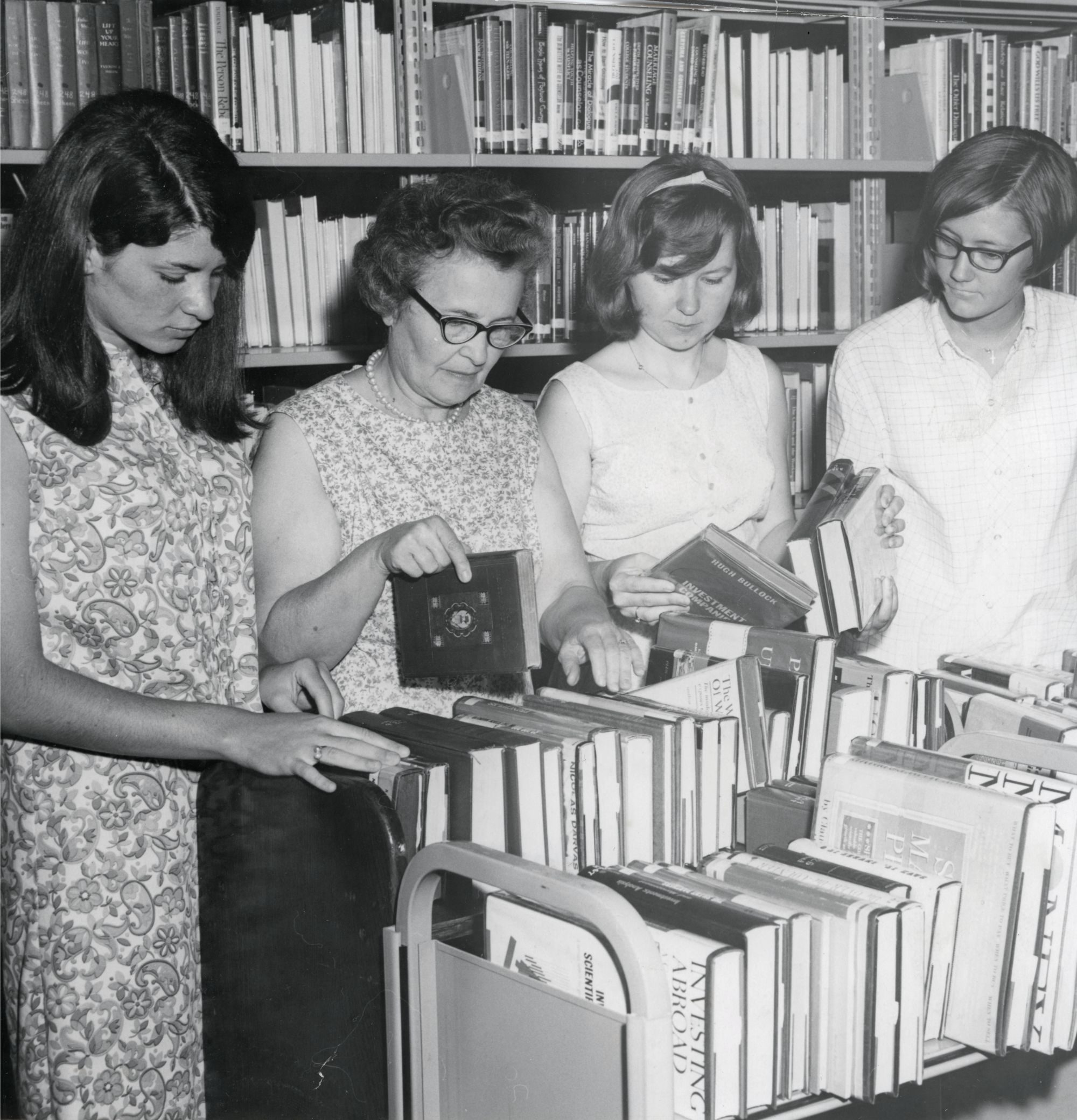This vintage black and white photograph captures a tight shot of four women in a library, either sorting or searching through books on metal library carts, which have distinctive U-shaped ends and two rows for holding books. Starting from the left, a young woman with dark hair, parted to the side, is wearing a sleeveless dress adorned with floral patterns. She is intently looking down at the books, with one hand resting on the cart and the other lightly touching a book. To her right, a slightly older woman with black glasses and a similar floral patterned sleeveless dress holds a book delicately between her thumb and index finger, the other hand resting flat on the books. Next, there is another young woman, also in a white sleeveless dress, with long brown hair cascading down as she examines a book held in her left hand, while her right hand holds two more books. On the far right, a woman with short brown hair, parted on the right, is wearing a white button-up blouse and black glasses, also focused on the books in front of her. Behind the women, rows of shelves filled with books create a scholarly backdrop, adding to the nostalgic atmosphere of the scene. All the women are dressed modestly, and the two on the left have similar floral dresses, emphasizing a harmonious yet individual presence in this timeless library setting.